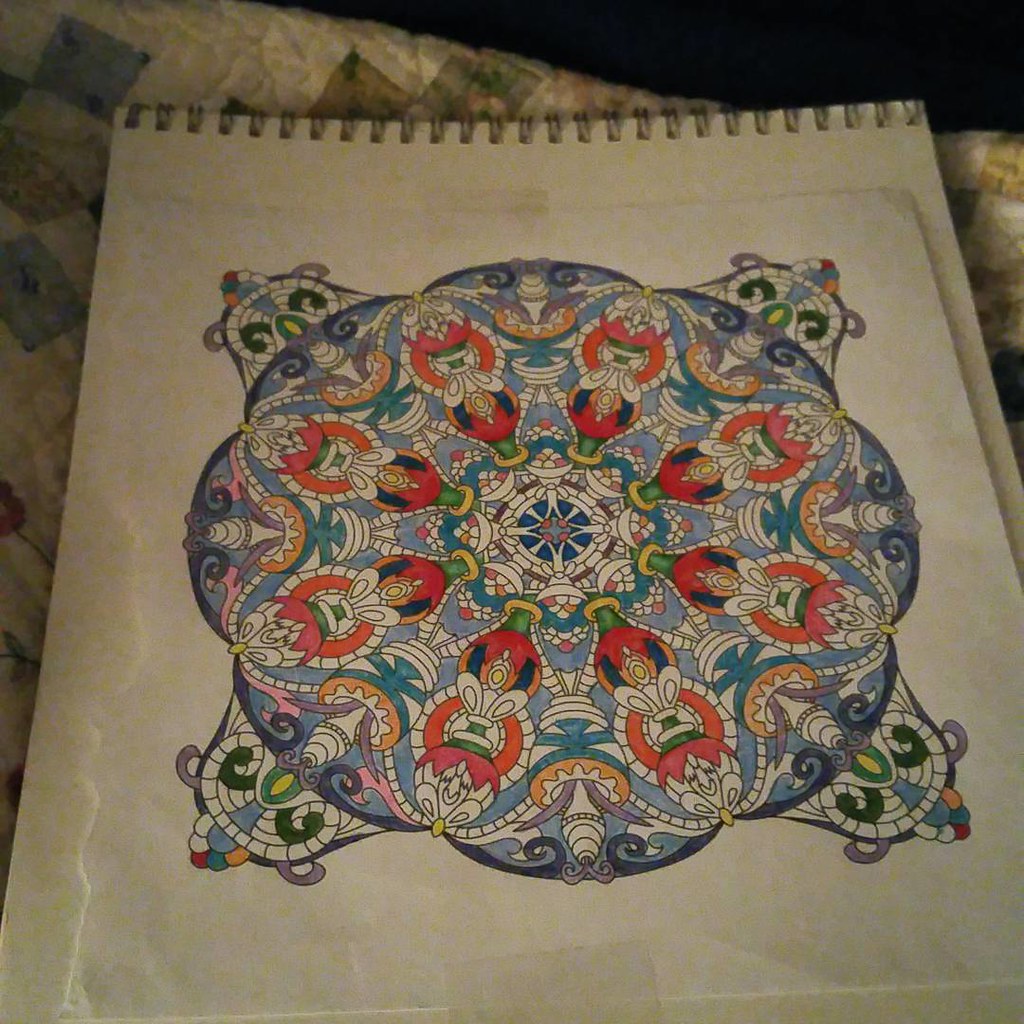A detailed color photograph showcases an elaborate pen and ink sketch that is colored in with a kaleidoscope of hues including green, red, orange, yellow, and dark blue. This intricate mosaic-like design, reminiscent of an ornate adult coloring book page, is taped to a sheet of white printer paper and positioned on a spiral-bound sketch pad. Prominently featured front and center, the sketch pad is placed atop an off-white, hand-stitched homemade quilt adorned with assorted blocks in blue and mustard yellow. The quilt's texture and patterns can be seen especially along the left side and upper left corner, with a dark brown background peeking through in one corner of the image.